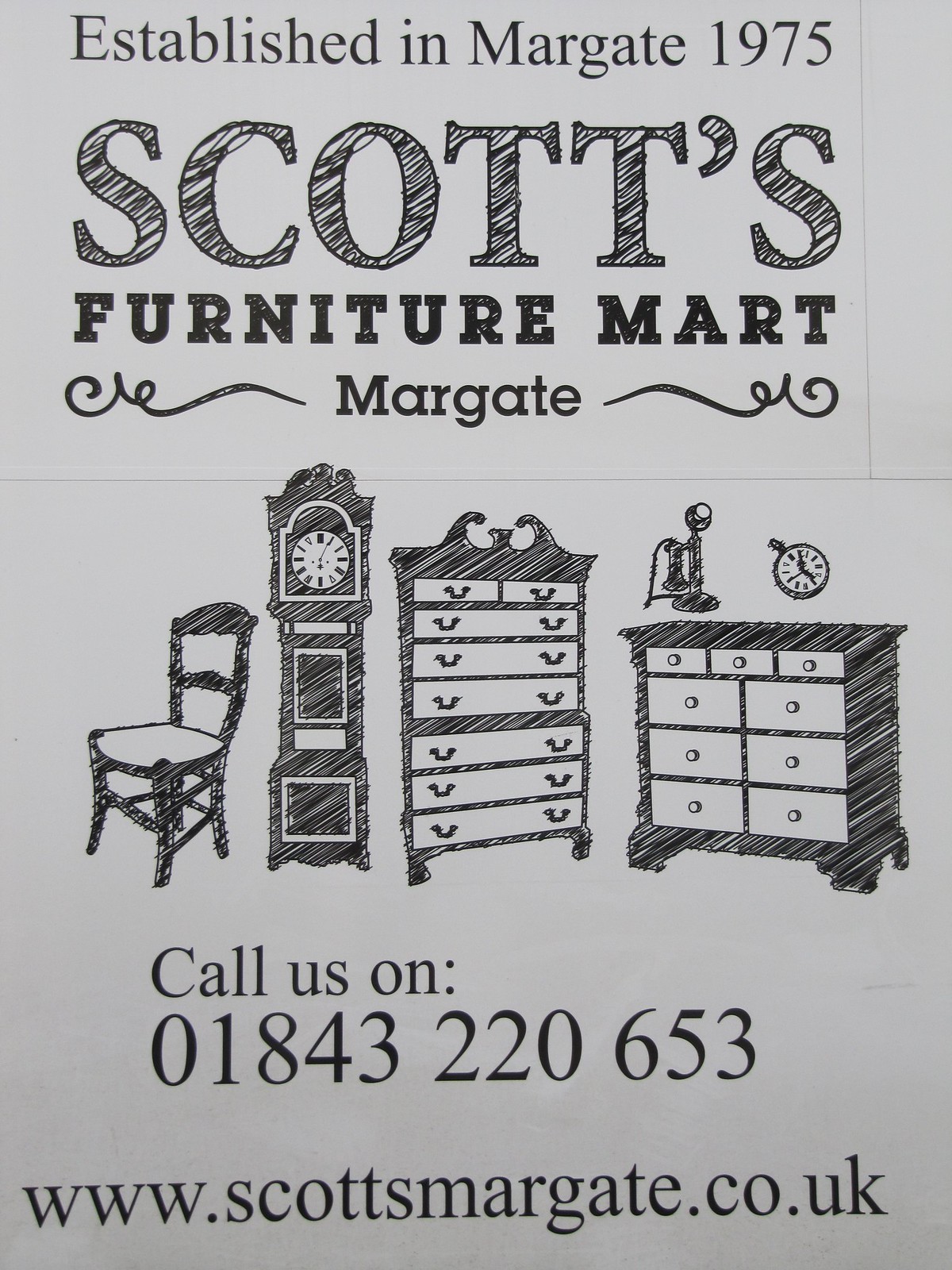This advertisement for Scott's Furniture Mart, established in Margate in 1975, has a vintage, hand-produced feel with a gray background and dark gray to black text. The top of the ad prominently features "Scott's" in a large logo, followed by "Furniture Mart" in smaller text, both flanked by decorative swirly elements around the word "Margate." Below this, detailed hand-drawn illustrations depict an array of furniture items including a chair, a grandfather clock, a chest of drawers, a bureau, an old-fashioned telephone, and a stopwatch. At the bottom of the ad, contact information is provided with the phone number 01843-220-653 and the website www.scotsmargate.co.uk. The overall appearance of the ad suggests a low-resolution, black-and-white scheme, possibly hand-drawn and lending it a quaint, nostalgic charm.